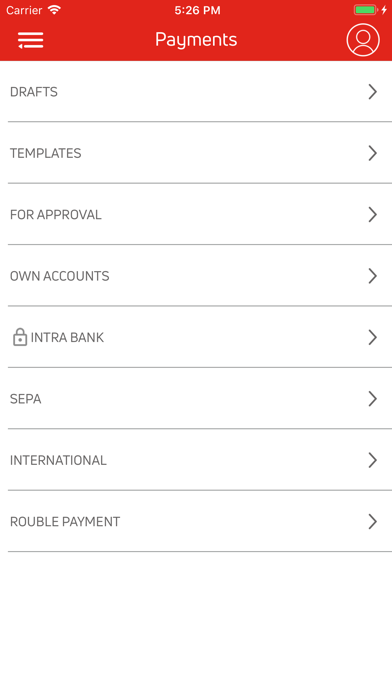The image appears to be a screenshot taken from a mobile phone interface, identified by the familiar status icons at the top. The banner area has a red background, with "Carrier" displayed in white text on the top left, followed by the Wi-Fi signal icon. Beneath this, there are three horizontal menu bars. Centered at the top, the time "5:26 PM" is shown in white, with "M White Payments" written below in larger letters. On the top right, a fully-charged green battery icon is visible, alongside a circular icon with a human silhouette representing account information.

Below the red banner, the main content of the screen consists of a list of menu options, each with an arrow pointing to the right. The first item is labeled "Dress," followed by "Templates." These are sequentially listed as "For Approval," "Own Accounts," "Intrabank" with a locked padlock symbol beside it, "SEPA," "International," and finally, "Ruble Payment." Each option is separated by faint gray divider lines, providing a clear and organized layout. The overall appearance suggests a streamlined user interface, likely for a financial or payment application.